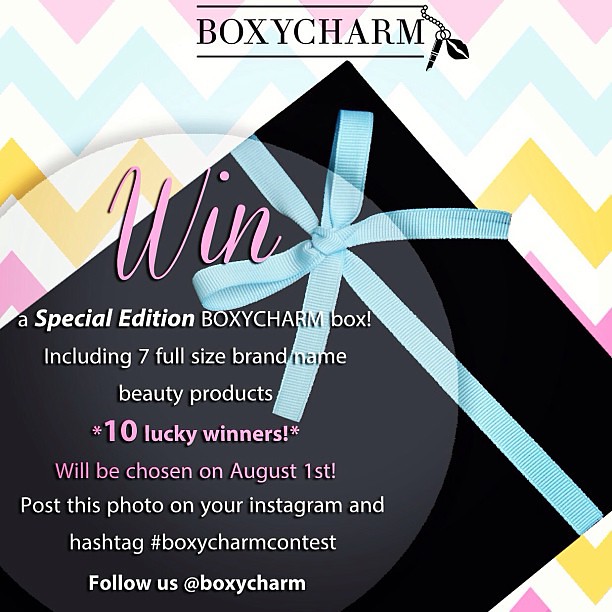The image is an advertisement for BoxyCharm. At the top, the name "BoxyCharm" is prominently displayed with horizontal zigzag lines in colors including pink, white, green, yellow, and blue creating a vibrant backdrop. To the right of the name, there's an intricate chain design featuring a pen and a mouth-shaped structure. Beneath this, in the center of the image, is a large black box adorned with a blue ribbon. The text on the box reads: "Wynn special edition BoxyCharm box including seven full-size brand name beauty products." Instructions for entering the contest are also included, stating that ten lucky winners will be chosen on August 1st. To participate, viewers are encouraged to post the photo on Instagram using the hashtag #BoxyCharmContest and follow @BoxyCharm.